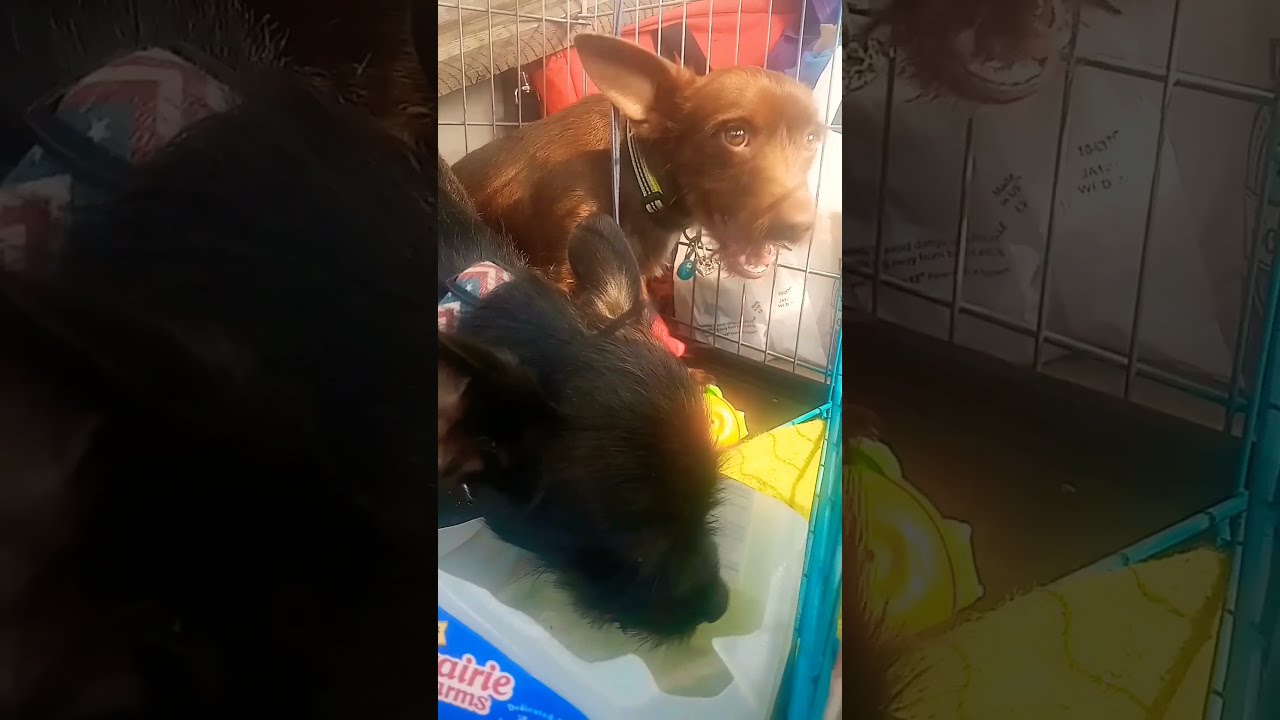In a faded and slightly blurry background, a full-size image showcases two dogs inside a kennel or cage. The front dog, black in color, has its head bent down, seemingly drinking from a container labeled "Prairie Farms." It sports a collar with an intricate design in different shades of orange and turquoise, resembling either an Indian or Chevron print. The black dog appears smaller in size compared to its companion and possesses ears that stick out. In the background, a larger, light brown dog looks off to the side with its mouth open. This brown dog has short fur, a neon green and black-and-white striped collar, and one pointy ear standing erect. Both dogs, looking somewhat skinny, appear as if they are about to be adopted, with their distinctly patterned collars contrasting their fur.